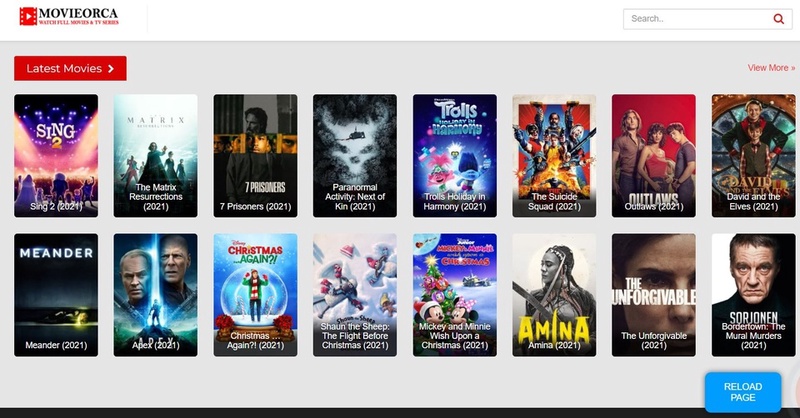On the Orca movie website, the latest selections of films are prominently displayed. Among the offerings are "Sing 2," "The Matrix Resurrections," "7 Prisoners" (2021), "Paranormal Activity: Next of Kin" (2021), "Trolls Holiday in Harmony," "The Suicide Squad," "Outlaws," "David and the Elves," and "Meander." For holiday enthusiasts, there's "Apex," "Christmas Again," "Shaun the Sheep: The Fight Before Christmas," "Mickey and Minnie Wish Upon Christmas," "Amina," "The Unforgivable," and "Border Town: The Mural Murders." The website presents each film with its captivating cover art, making it easy to decide what to watch next. It's a perfect setup for a cozy movie night, ensuring you can never go wrong with the choice of films available.